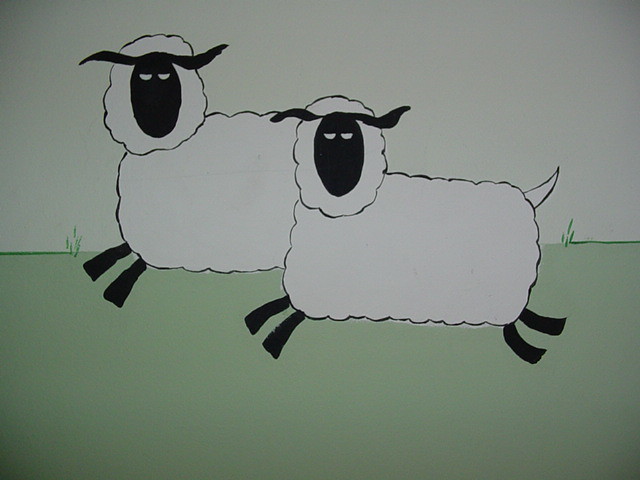This image features a simple yet detailed drawing of two energetic sheep, depicted as running or jumping across a muted green field. The bottom half of the image showcases the green field, transitioning into a pale gray sky in the upper half. On both the left and right sides, about an inch inward, there are small strokes of green extending into the gray area, suggesting sparse blades of grass.

The sheep, centrally located and positioned more towards the top of the frame, possess white, fluffy bodies and short, white tails. Their legs and faces are black, with the latter featuring distinct, simplistic characteristics: black ears, two white slit-like eyes without pupils, and faces that gaze directly at the viewer. The sheep's forward-leaning postures, with front legs extended and back legs trailing, convey a sense of motion and liveliness. The absence of intricate details on their bodies, combined with their overall stylized and curved outlines, adds to the drawing's minimalist charm.